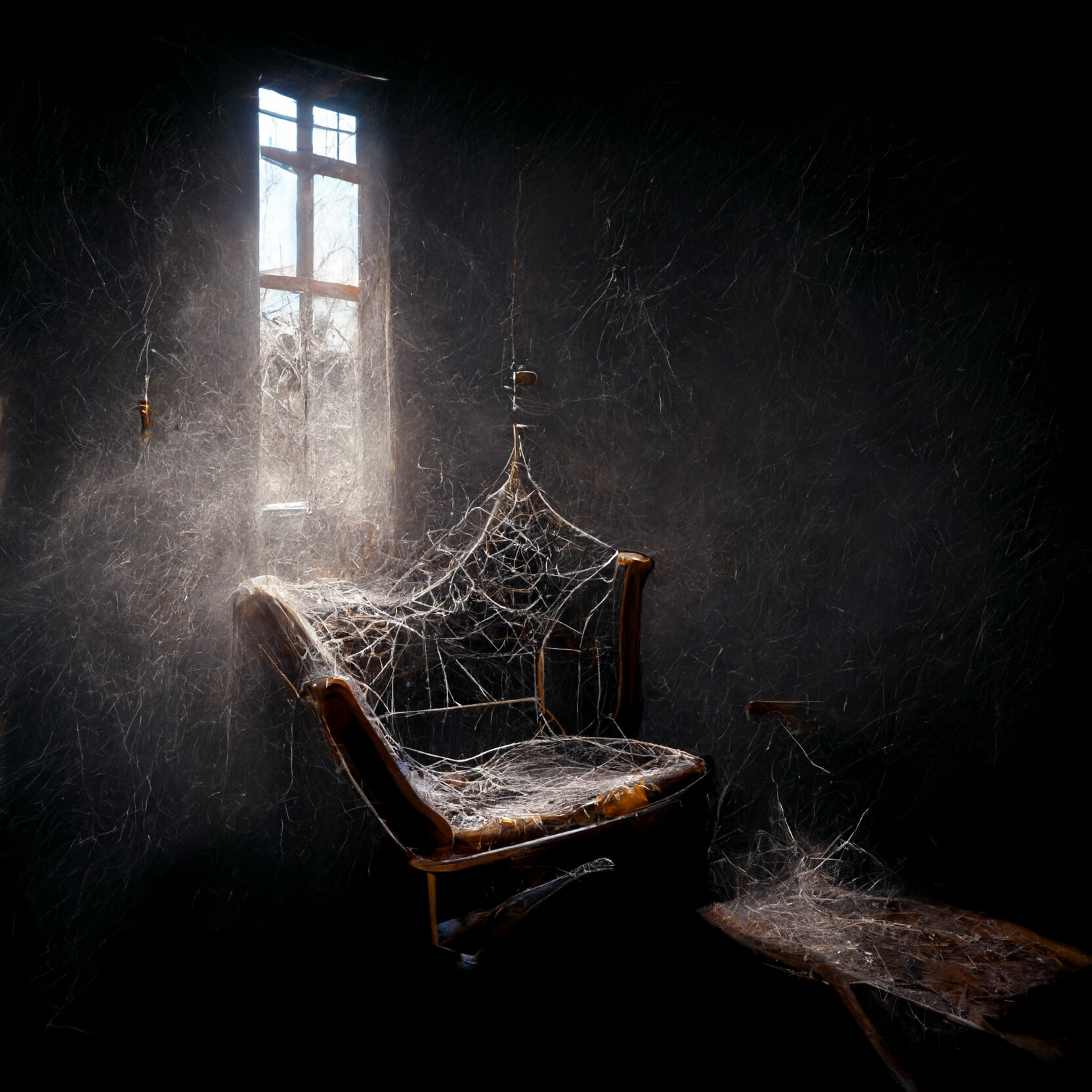The image depicts a dark, almost black room inside what seems to be a home. Light filters in through two large windows, illuminating the blue sky and a hint of a bush outside. Inside, the scene is dominated by numerous white cobwebs that drape across various objects, giving the room an eerie atmosphere. A brown chair, equipped with a silver lever for reclining, stands prominently and is heavily covered in cobwebs. Nearby, there is a brown headboard and a bench, both also ensnared in cobwebs. A small light string hangs on the left-hand side, adding a faint glow to that area. Cobwebs dangle from the ceiling, and the overall space is shrouded in dust and fog, enhancing the abandoned and ghostly feel of the setting.